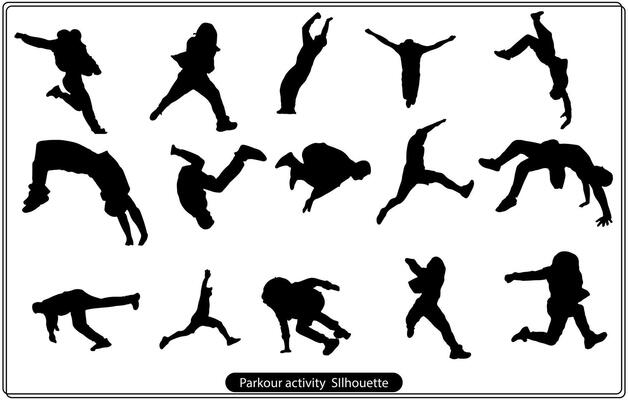The image features a white rectangular background with a thin black border and showcases a series of 15 black silhouettes arranged in three rows of five. Each silhouette captures various dynamic poses representative of parkour movements, such as jumping, running, and landing. Above these illustrations, the phrase "Parkour Activity Silhouette" is displayed in white letters within a long, narrow oval with curved ends. The silhouettes depict a single figure performing a sequence of moves, demonstrating the acrobatic nature of parkour, typically executed in an urban environment. This detailed illustration appears to be either an instructional guide or an artistic poster, ideal for parkour enthusiasts to visualize and celebrate the diverse maneuvers involved in the activity.